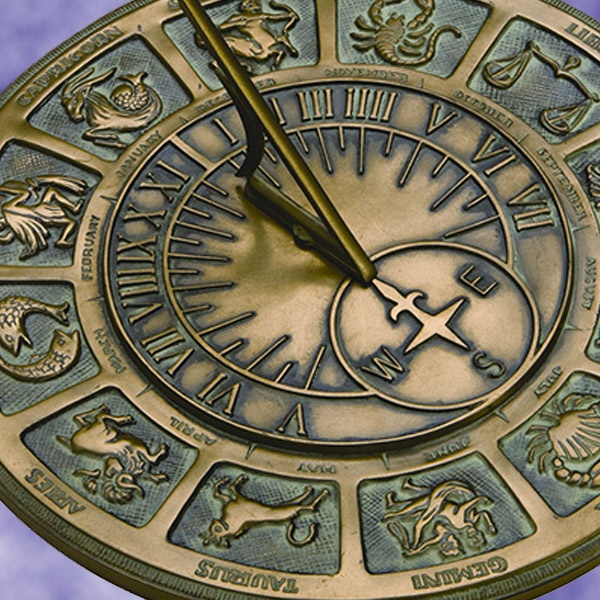The image depicts a square-shaped, intricately detailed bronze sundial, approximately five inches in both height and width. The background is adorned with blotches of purple and lavender, particularly visible in the four corners. The sundial itself is slightly off-centered, extending beyond the top and bottom left and right sides of the image.

The outer rim of the sundial is embellished with images of zodiac signs and their corresponding names, such as Gemini, Taurus, Aries, Pisces, and Capricorn. At the bottom of the image, Gemini, Taurus, and Aries are prominently displayed. Other zodiac characters, like the centaur, scorpion, and scales, are also visible, with partial images of Libra and a man near Pisces noted.

Beneath the zodiac signs, the inner ring of the sundial indicates the months of the year, with Roman numerals marking the hours. Notably, the dial is currently pointing at July, aligning with the Cancer sign (noted as the crab). At the center, a raised circle indicates the four cardinal directions: North, South, East, and West.

The sundial, made of dark brass with black etching around each digit and figure, has a shiny finish. The central gnomon, part of the sundial that casts the shadow, is marked with these directional points, creating a cross-like shape within the center circle.